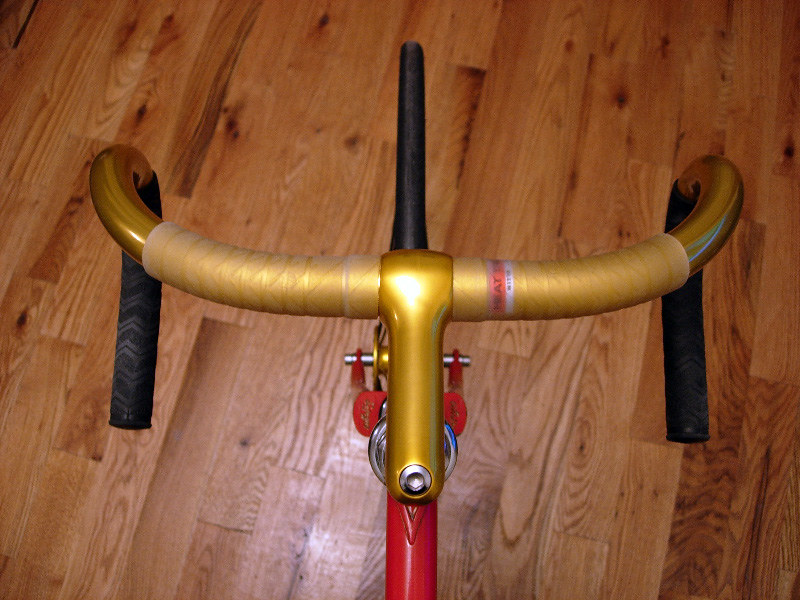The image is a top-down shot of a bicycle positioned on a clean, shiny hardwood floor. The focal point is the front section of the bicycle, prominently featuring golden handlebars with black grips characterized by some lined patterns. The red frame of the bike is also visible, contrasting sharply with the golden and black elements. Although the front wheel is suggested to be just out of view or barely visible, its presence is implied beneath the visible portions of the bike. This indoor photograph suggests that the bike might be new or has not yet been taken outside. No gear shifts are visible on the handlebars. The lighting from above reflects off the floor, contributing to the clean and polished appearance of the setting.